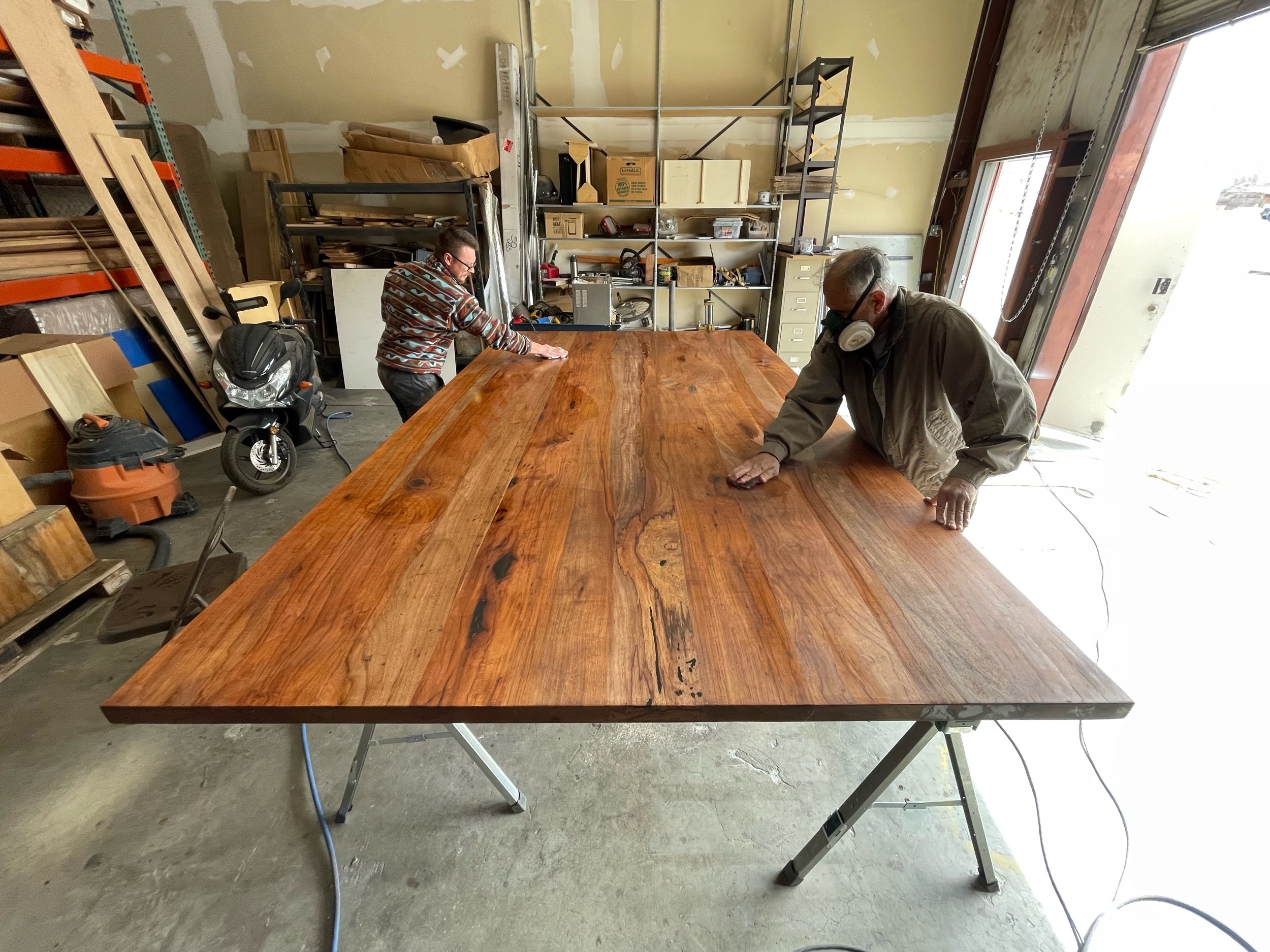In a well-lit garage with a commercial-style metal rolling door, two men are intently working on a large wooden plank, likely meant for a dining room table. The man on the right, who has gray hair and is donning a loose-fitting gray jacket coupled with a ventilation mask, appears to be sanding the wood. The other man, standing to the left, is wearing glasses and a blue and brown sweater. He seems to be rubbing a stain into the now slightly shiny surface of the wood. The surroundings include numerous shelves cluttered with woodworking equipment and materials. In the back left corner, a black motorcycle is parked beside an orange shop vacuum.